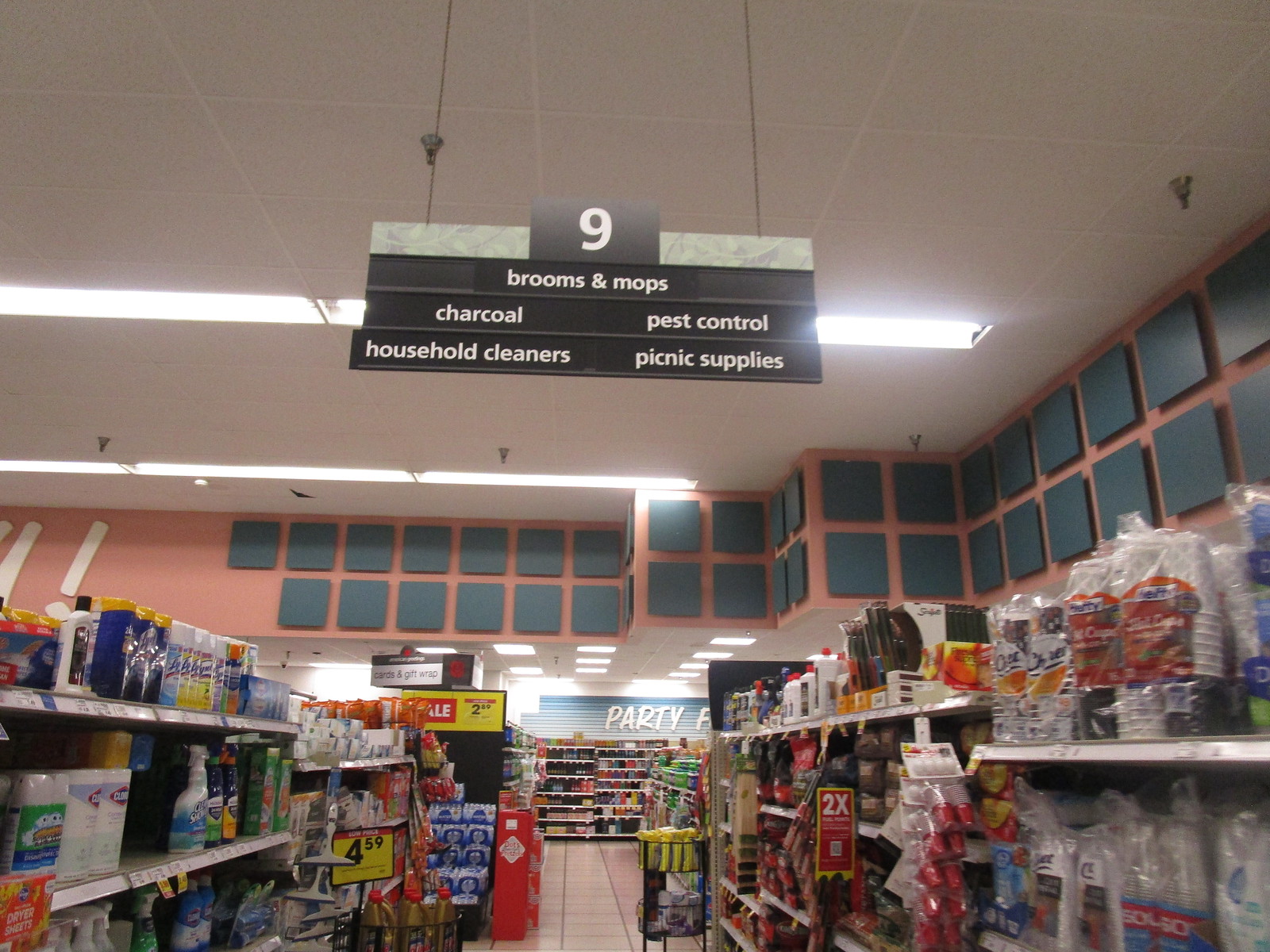A colorful, horizontal photograph captures a store aisle with a prominently displayed sign indicating "Aisle 9" at the top. The sign lists various product categories, including brooms and mops, charcoal, pest control, household cleaners, and picnic supplies. The sign itself is predominantly black and white, accented with a subtle green border.

The aisle is stocked in accordance with the sign, featuring an array of household cleaning products like Lysol, and stacks of styrofoam cups among other items. Towards the back of the aisle, another sign labeled "Party" can be seen, though it's unclear if it refers to party supplies specifically. 

The store's flooring is a distinctive salmon pink, which contrasts with the marble white ceiling, adding an interesting visual dimension to the scene. The aisle appears spacious, providing ample room for shoppers to navigate.